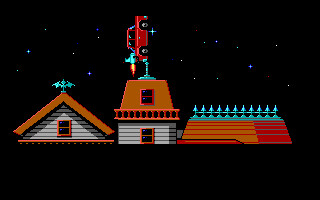This computer-generated image depicts the upper portion of a house with intricate details. The house features a distinct red roof and gray siding. Atop one of the roofs stands a weather vane shaped like a bird with visible wings. The adjacent roof on the right side hosts a line of green shapes resembling birds perched in a row. Centrally located is a prominent gable, known as a widow's peak, adorned with detailed red molding. Additionally, all the windows are trimmed in red. A unique element in this scene is a car situated on this particular roof, appearing as though it is about to take flight. The car shows signs of ignition, with vibrant red, yellow, and orange flames bursting from its rear, giving the impression of an imminent takeoff.